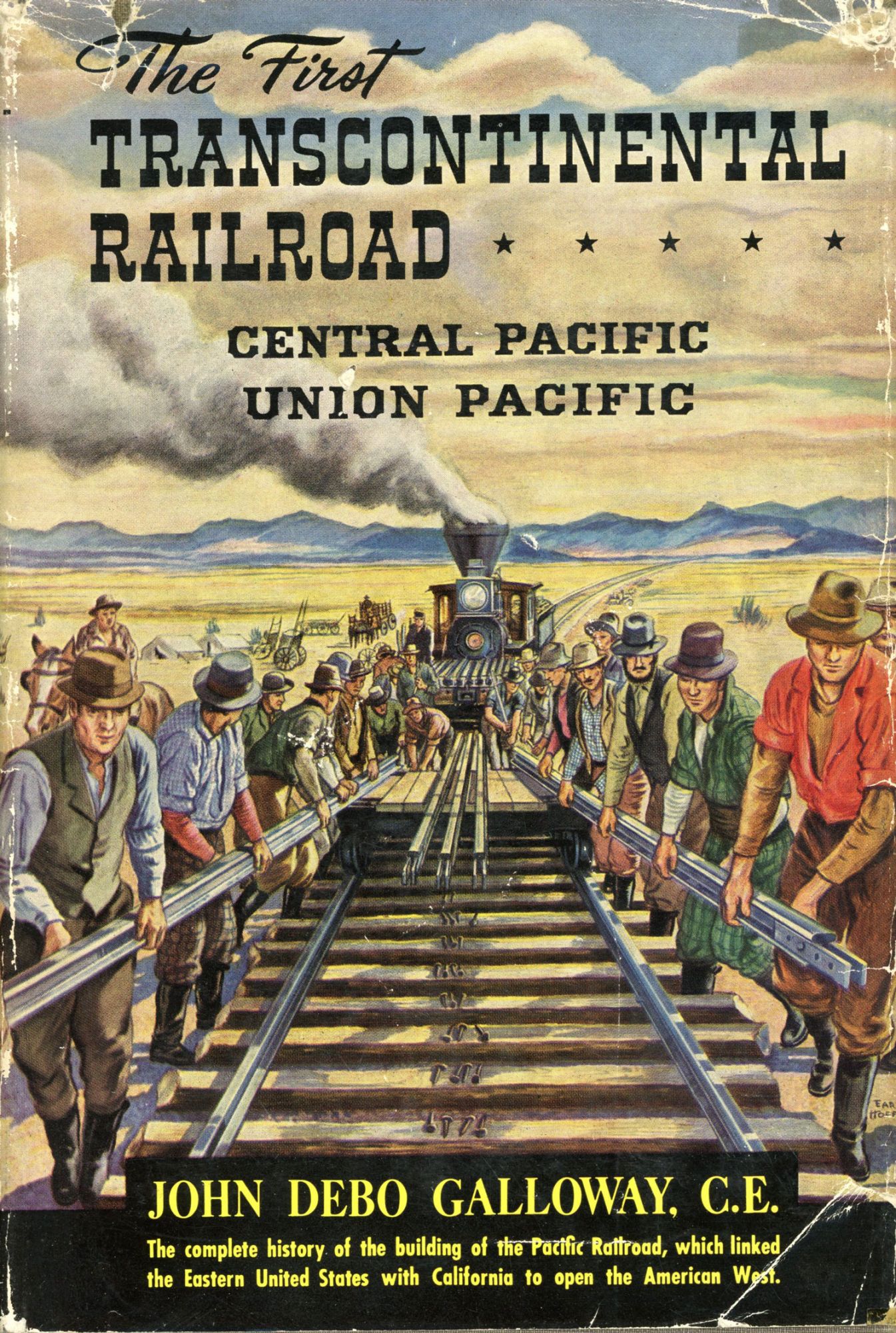This artistic poster depicts the monumental construction of the first Transcontinental Railroad, specifically the Central Pacific and Union Pacific lines. Centered in an expansive, desert-like landscape, the scene captures the momentous effort of men laying railway tracks. The men, donned in work shirts of various colors such as light reds, greens, blues, and grays, and wearing caps, are positioned along the tracks, placing heavy metal rail lines. A steam locomotive, emitting smoke, advances along the newly laid tracks, symbolizing progress. Above the image, the caption reads "The First Transcontinental Railroad, Central Pacific, Union Pacific" in bold black letters. Blue mountains rise in the distant background, adding depth to the vast, unsettled plains. At the bottom of the poster, in yellow text, it credits John Deboe Galloway, C.E., and highlights "The Complete History of the Building of the Pacific Railroad," celebrating the connection forged between the eastern United States and California, thus opening the American West.